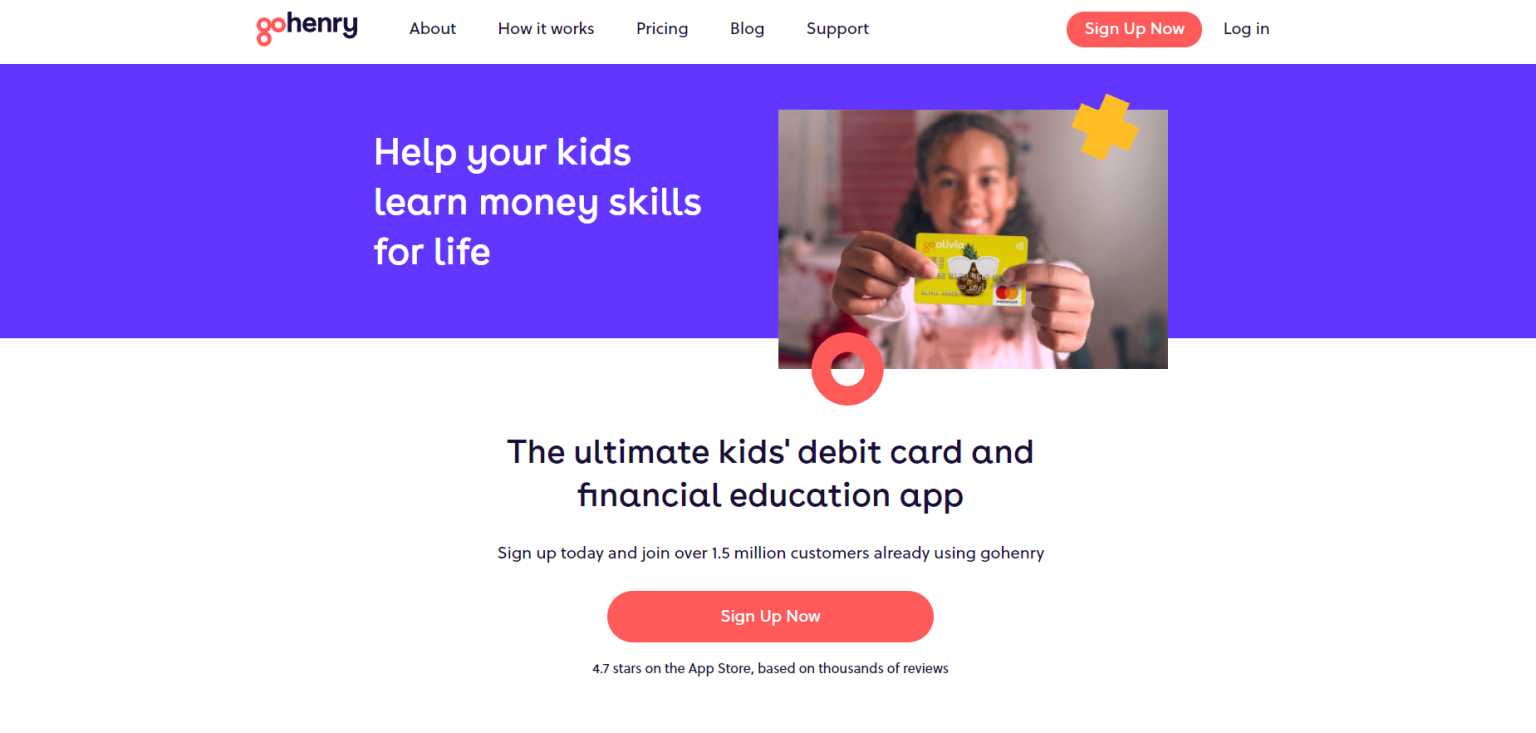This screenshot captures the homepage of the GoHenry website. The top left corner prominently displays the GoHenry logo, with "Go" in orange and "Henry" in black. Adjacent to the logo, the navigation bar spans from left to right, featuring tabs labeled About, How It Works, Pricing, Blog, and Support. At the far right end of the navigation bar, an eye-catching orange button invites visitors to "Sign Up Now," followed by a "Log In" option.

Just below the navigation bar is a vibrant purple horizontal stripe, adorned with white text on the left that reads, "Help Your Kids Learn Money Skills for Life." To the right, an image of a young girl holding up a yellow card with a brown symbol (likely money-related) draws attention. The image also includes decorative elements: an orange circle in the top left and a yellow "X" in the top right. Immediately beneath this section, bold text announces, "The Ultimate Kids Debit Card and Financial Education App," succinctly conveying the website's purpose of providing financial education and tools for children. The overall design and content strongly suggest that GoHenry is a kid-focused financial app aimed at teaching money management skills.